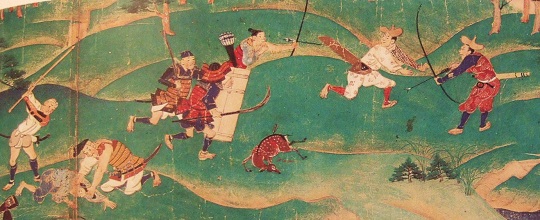The image appears to be an ancient Asian artwork, likely from Japan or China, featuring traditional scenes of conflict and activity. The central focus includes multiple figures with black hair, adorned in old-fashioned attire, primarily in shades of red and white. The clothing suggests historical or traditional Japanese influence. The scene depicts a tumultuous moment, possibly a battle, with individuals shooting crossbows and engaging in combat. A deer is seen slumped over amidst vibrant green hills and trees in the background, which have a distinctive halo-like glow. The palette is rich and varied, dominated by green and blue hues, with significant splashes of red, orange, brown, and white. Even though the figures are somewhat distant, the overall scene is vibrant and dynamic, encapsulating a moment of intense action in a lush, colorful setting.